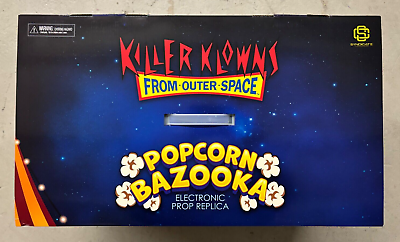The image depicts the front of a product box designed with a space-themed background, featuring a bluish center transitioning to black filled with white stars. Dominating the top is the title "Killer Klowns" in a scary, red font, with "Klowns" notably spelled with a 'K'. Below this, a prominent yellow banner outlined in red frame displays the phrase "From Outer Space" in blue text. Beneath this banner, the product name "Popcorn Bazooka" appears in bold yellow letters, surrounded by images of both white and brown pieces of popcorn. Directly under the product name, the label "Electronic Prop Replica" is written in white font. Additional details include a plastic handle at the top, some red and orange decorative bands in the lower-left corner, a logo with the letters "SC" in the upper right, and a product warning in the upper left corner.